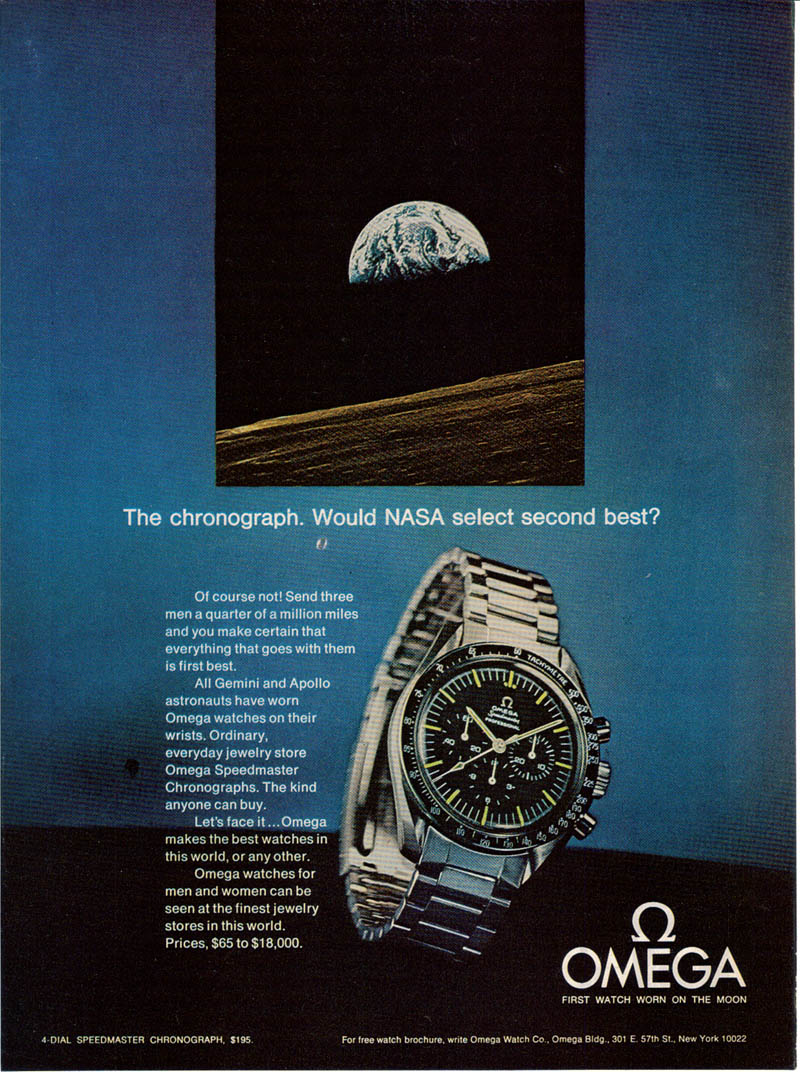This vertical magazine advertisement features the Omega Speedmaster chronograph watch. The top half of the ad showcases a stunning image of Earth seen from space, resembling a downturn half of a line on a black background. The Earth hovers above a black surface that transitions into a dark blue wall, which gradually lightens towards the top. Below this image, a bold line of white text on the blue background reads, "The chronograph would NASA select second best?" Below this, there's an emphatic response: "Of course not. Send three men a quarter of a million miles and you make certain that everything that goes with them is first best. All Gemini and Apollo astronauts have worn Omega watches on their wrists." The ad highlights that these are the Omega Speedmaster chronographs — the kind anyone can buy at an ordinary jewelry store. Further text emphasizes the brand's prestige, stating that Omega makes the best watches in the world or any other and that these watches for men and women can be found at the finest jewelry stores, priced between $65,000 to $18,000. In the bottom right corner, the iconic Omega logo is displayed with the tagline, "Omega, first watch worn on the moon." Lastly, a close-up of the elegant gray metal watch with a black face is showcased, seemingly floating against the dark background.